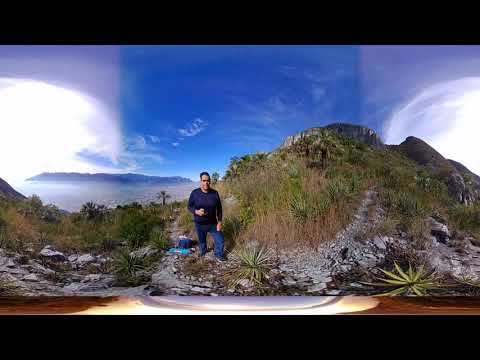A middle-aged man is posing for the camera while on a nature hike. He's dressed in a blue shirt and blue jeans, standing amidst rocky terrain mixed with pebbles, grass, and cacti-like shrubbery. It’s a bright, sunny day with partly cloudy skies, casting a beautiful light over the scene. In the distance, you can see hills topped with brush and what seems to be a vast ocean or large body of water, creating a stunning landscape reminiscent of an island with water separating it in the background. The man, likely enjoying his solo adventure, seems prepared with a backpack and possibly holding a beer in his right hand, with a box or some sort of equipment at his feet. The panoramic image captures the serene and remote atmosphere of his hike, emphasizing the tranquility of being surrounded by untouched nature.